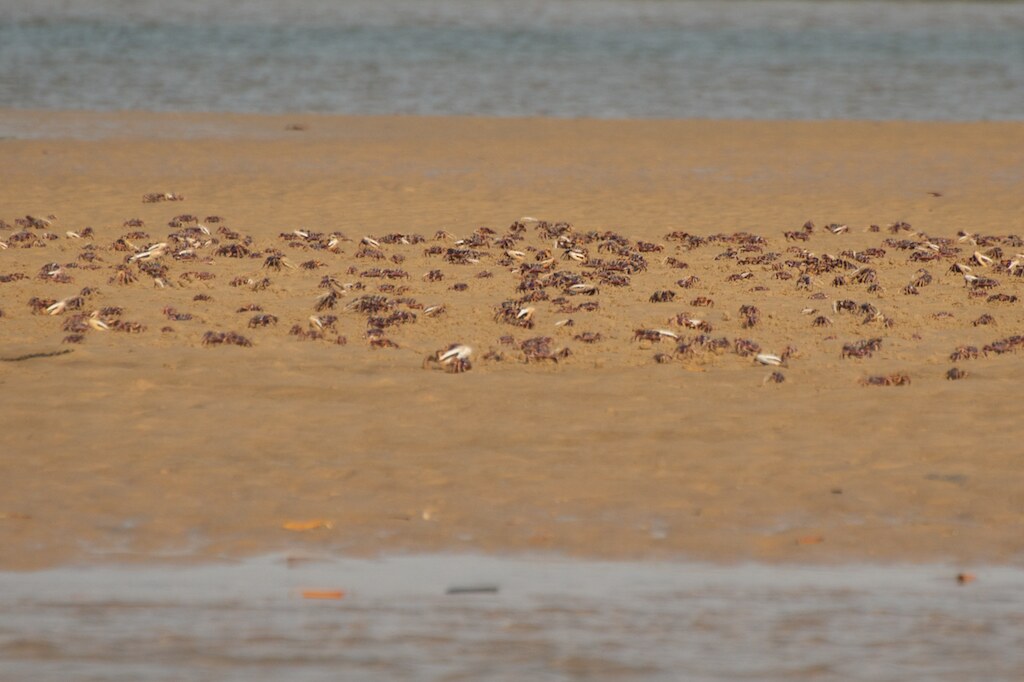The photograph captures a tranquil sandbar surrounded by calm, shallow waters, visible both at the top and bottom fifths of the image. The scene exudes a sense of serenity, underscored by the absence of significant waves. In the foreground, assorted sticks and debris float, adding to the natural ambiance. The central expanse of the sandbar is dotted with small, brownish objects that closely resemble a sizable colony of crabs. These creatures, numbering between 50 and 100, display grey-striped or possibly greenish shells with distinctive pincers. This serene, isolated sandbar offers an ideal habitat for these crabs to thrive, likely serving as a breeding ground protected from the ocean's currents.